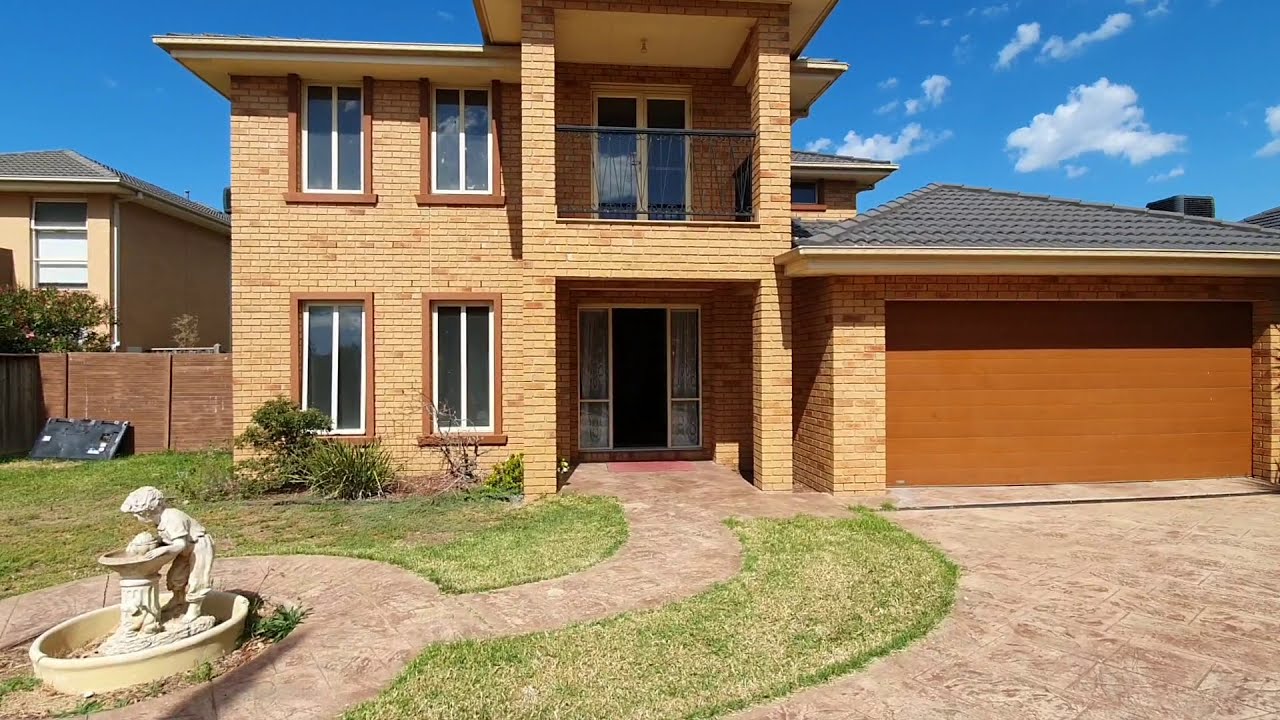The image depicts a charming two-story brick house with predominantly light yellow bricks interspersed with darker brown ones. The house features tall, two-panel windows with brown trim on both the top and bottom floors on its left side. To the right is the entrance, marked by a dark brown door flanked by slender rectangular windows with white trim. Above the door, a balcony with a black metal railing and a sliding glass door with white trim peeks out from beneath the roof’s overhang.

The front door opens onto a walkway made of rock-colored panels that branches left into a circular path around a dry, ornamental fountain resembling a young boy leaning forward. The walkway also extends towards a medium brown garage on the right side, which is topped with an arched roof adorned with black tiles. The driveway leading up to the garage is composed of smooth pavers in beige and terracotta tones, complementing the house's overall aesthetic.